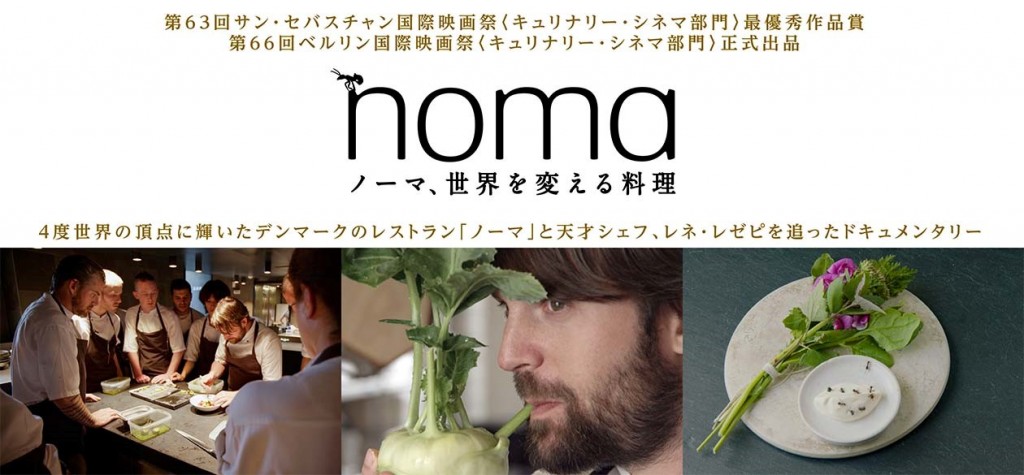This advertisement for a restaurant prominently features the name "Noma" in English, with an insect perched on the letter "N," and is surrounded by Japanese writing above and below. The layout includes a panel at the bottom with three distinct images: 

1. On the left, a group of chefs in white shirts and brown aprons work collectively in a kitchen around a countertop filled with various plates and containers. One chef is actively preparing a dish while others observe.
2. In the middle, a Caucasian man with medium-length brown hair and a beard sips from a stylish drink through a straw inserted into a vegetable base.
3. On the right, a blue surface holds a plate garnished with pink flowers and either bok choy or another vegetable, with a smaller white plate on top containing a creamy dish, possibly garnished with ants.

The advertisement uses a mix of black and gold text for the Japanese characters, set against a background highlighted by a predominantly green and white color palette. This eclectic presentation aims to entice potential diners by showcasing the restaurant's unique offerings and culinary artistry.